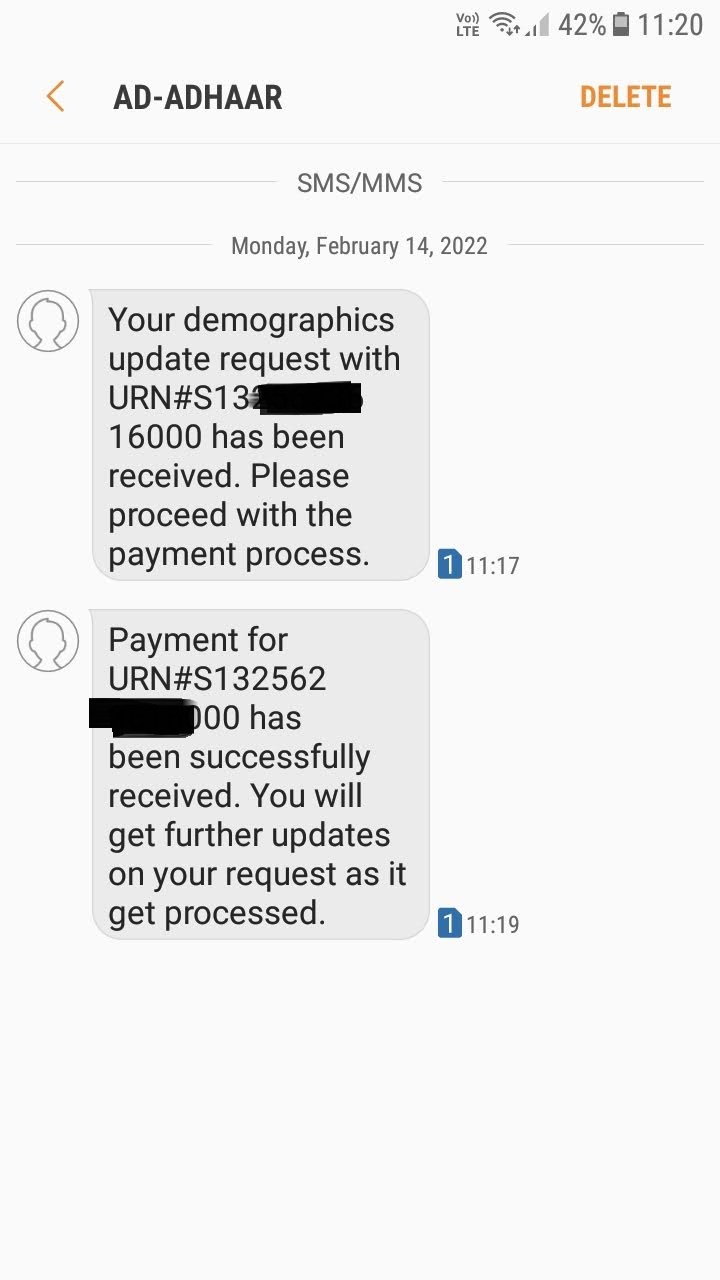Screenshot of Mobile Messaging App Interface

The image is a screenshot from a mobile device displaying a message app. The sender's name, "Ad-Adhaar" (A-D dash A-D-H-A-A-R), appears at the top with a left-facing arrow icon indicating a back button to the left of the name. To the right, there is an orange "DELETE" text in all caps. 

In the top right corner of the screen, various phone interface icons are visible, including indicators for LTE, Wi-Fi, mobile signal strength, and battery level, which is at 42%. Additionally, the time displayed is 11:20.

The main content of the screenshot shows a conversation thread labeled "SMS/MMS." The date "Monday, February 14, 2022" is noted below this label. A default outline avatar is shown where the sender’s profile picture would typically be.

The screenshot captures two messages from the sender:

1. The first message, sent at 11:17, reads: "Your demographics update request with URN #S13****** has been received. Please proceed with the payment process."
2. The second message, sent at 11:19, states: "Payment for URN S13****2562****** has been successfully received. You will get further updates on your request as it gets processed."

Certain parts of the URN (Unique Reference Number) and other sensitive information have been redacted for privacy. The image effectively captures the device's messaging interface and the details of the communication with "Ad-Adhaar."